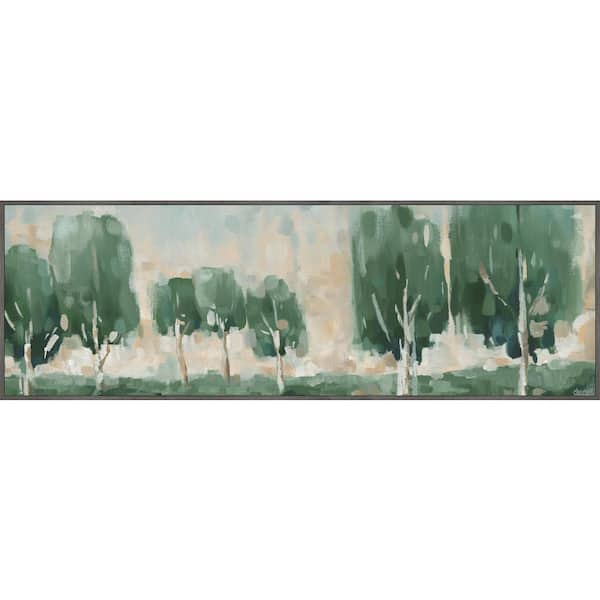The image depicts a simple yet striking watercolor painting, presented in an elongated rectangular landscape orientation, framed neatly in either a dark brown or black frame. This impressionistic artwork features a serene assembly of approximately seven trees, portrayed with blotchy, fluid brushstrokes that evoke the delicate translucency characteristic of watercolors. The trees, with their circular green canopies and long, beige trunks, stand in varied sizes—two tall ones anchoring the left side, three shorter ones clustered next to them, and two more prominent ones on the far right. The background blends an array of colors—shades of greens, pinks, beige, and hints of orange—creating an impressionistic scene with low-lying green hills. The sky, painted in soft, warm tones of beige and pink, offers a pleasing contrast to the greens of the trees, enhancing the tranquil, dream-like quality of the mural.